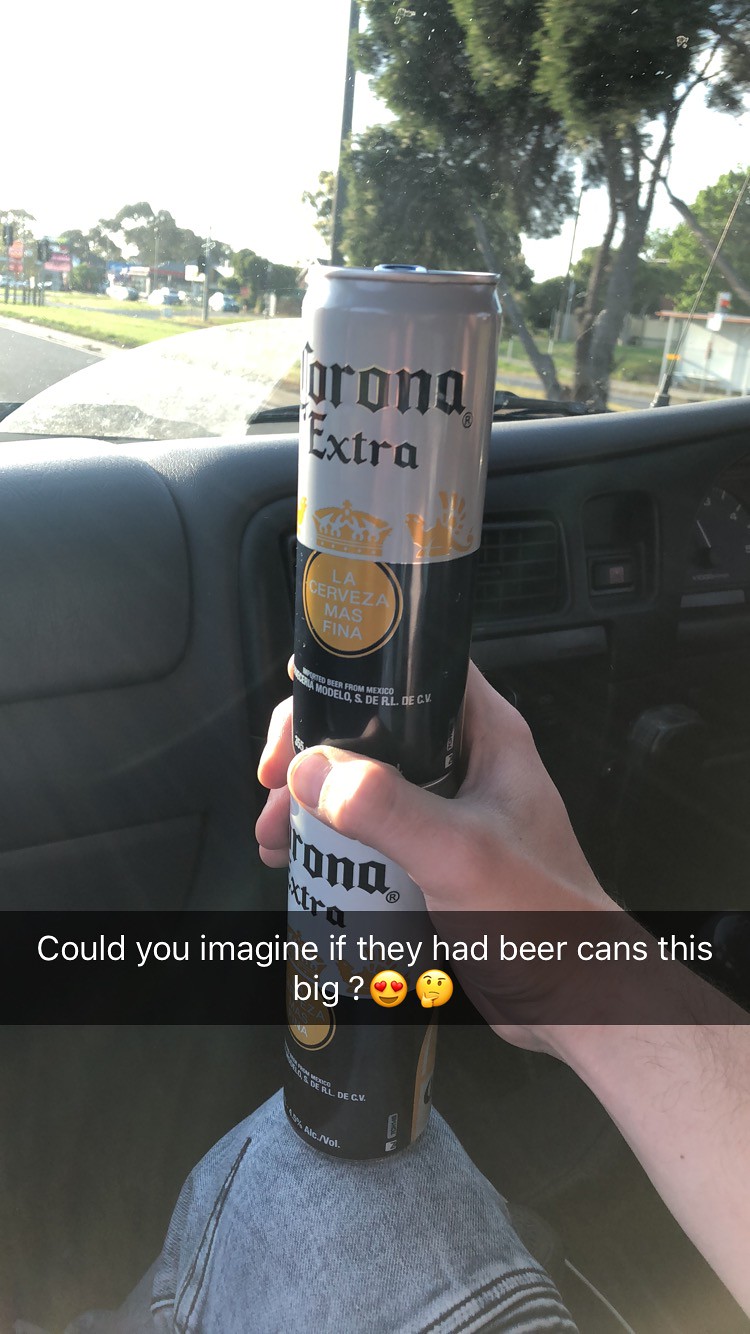This photograph, likely taken on a phone and shared on social media, including platforms like Instagram or Snapchat, captures a playful scene inside a car. A presumably Caucasian man, dressed in blue-gray jeans, sits in the driver's seat with his hand, which is slightly hairy, carefully propping up two stacked, skinny cans of Corona Extra beer on his knee. The cans, featuring a white top with the gold Corona logo and a blue bottom, are almost perfectly aligned, making them appear as a single, oversized can.

A black textual overlay, approximately two-thirds to three-quarters down the image, humorously reads, "Could you imagine if they had beer cans this big?" followed by a heart face emoji and a thinking emoji, hinting at the man's amused and contemplative mood. 

In the background, the car's interior is mostly black, with visible air vents and a gray dashboard. Through the clear windshield, a sunny scene unfolds with a road bordered by grass and trees, including a large tree on the right side and more trees in the distance under a pale sky. The image captures a light-hearted moment, contrasting the everyday interior of a car with the whimsical stacking of beer cans.